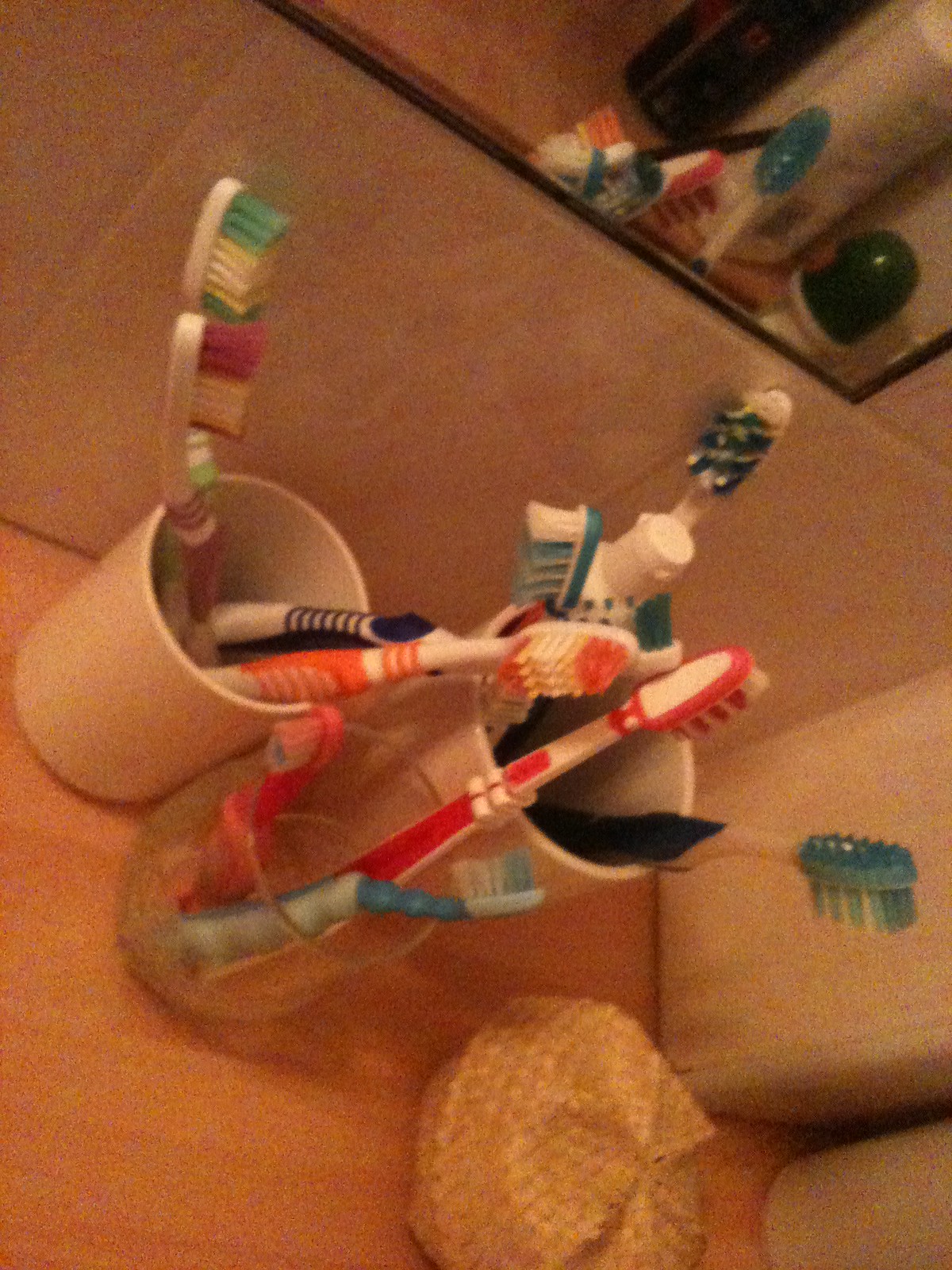The photograph displays a light brown wooden bathroom counter populated with three cups holding a range of toothbrushes. The image is slightly turned to the right, giving a comprehensive view of the scene. In the upper right corner, a part of a mirror with a black outline is visible, reflecting the multitude of toothbrushes.

On the left, a white ceramic cup holds four toothbrushes, featuring green, beige, and purple bristles, in a striped pattern. Specifically, there are green, beige, and purple toothbrushes, with a consistent alternating bristle design. The middle clear cup, shorter in stature, contains three toothbrushes: two small children’s brushes, one pink and one blue, alongside an adult red toothbrush. The cup's transparent nature allows easy visibility of the switches in bristle colors—light orange, white, and blue.

The rightmost cup, also white ceramic, holds three diverse toothbrushes. Among them is a toothbrush with a dark blue handle and blue to light blue bristles, transitioning to white. Another toothbrush features a darker blue with alternating white and blue bristles. There’s also a short green toothbrush visible.

On the counter, set against a backdrop of beige-tiled walls, there is a cylindrical object wrapped in beige, tan, polka-dotted fabric, possibly holding soap. Completing the ensemble are two partially shown containers—a large square white one and another cylindrical white container.

This vivid composition captures the organized chaos of a family’s array of dental hygiene tools against the serene backdrop of a typical, cozy bathroom space.